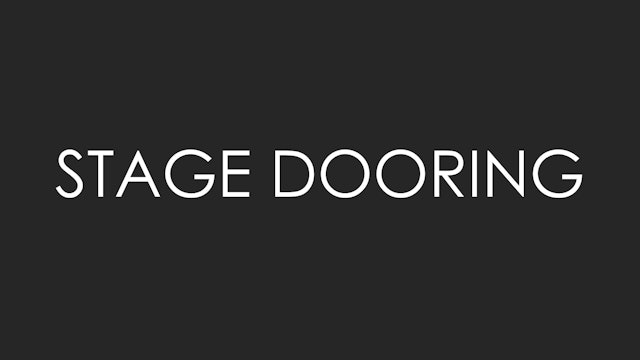In the rectangular image, which is approximately twice as wide as it is tall, there is a minimalistic yet striking design devoid of any objects except for text. The entire background is a deep, solid black, creating a stark contrast with the pure white, all-uppercase text that reads "STAGE DOORING." This text is centrally positioned both vertically and horizontally, running from left to right but stopping about an inch from both sides, ensuring it does not touch the edges. The simplicity and style of the text, reminiscent of Helvetica, suggest it could be used as a sign in a variety of professional or formal settings, such as a stage, conference center, hotel, gallery, or museum. The overall aesthetic is clean and functional, clearly intended to convey a message with no additional graphic elements.